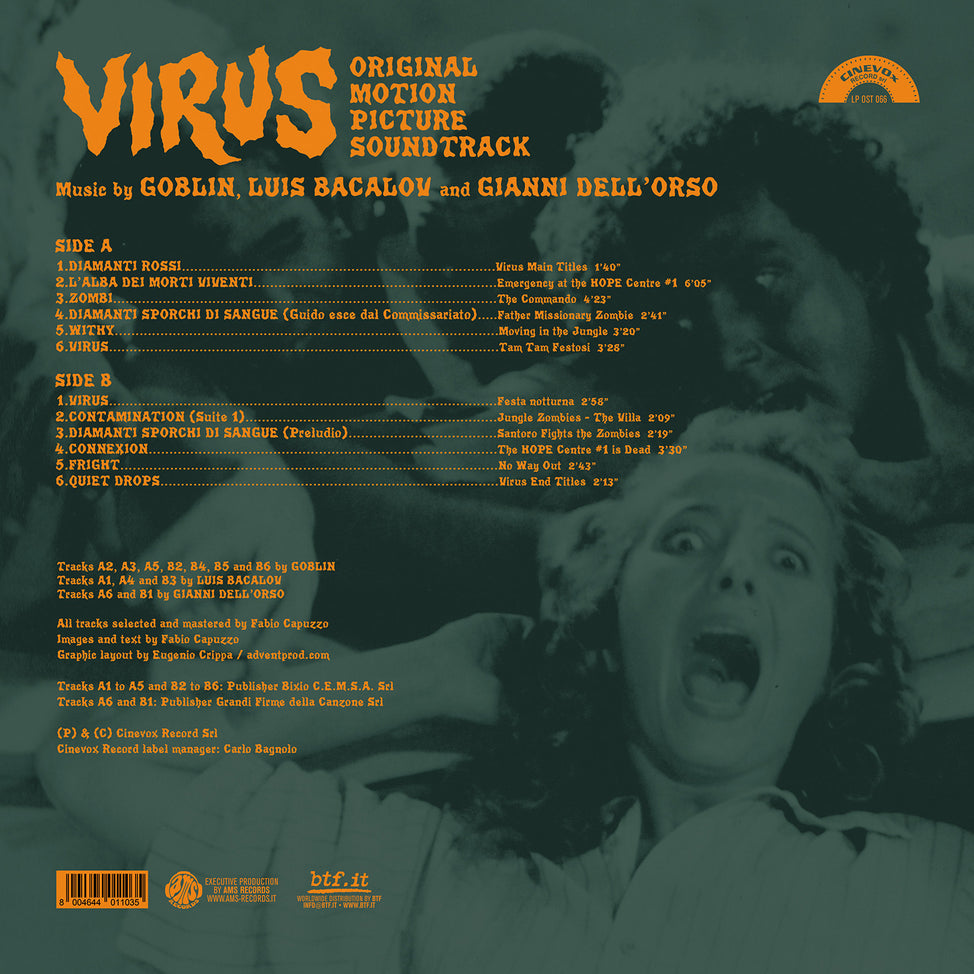This image serves as the liner art or back cover for the "Virus" original motion picture soundtrack CD. The primary visual element is a dark, blue-tinged background featuring a striking scene from the film. In the bottom right corner, a woman with long, curly hair is depicted screaming in fear, her eyes and mouth wide open, and her right hand held up behind her head. Above her, a man with darker skin and short, curly hair gazes off to the left, while another man with short dark hair looks down and to the right, reaching an arm towards the woman.

The detailed orange text overlaying this dramatic scene reads "Virus, original motion picture soundtrack" followed by "music by Goblin, Luis Bacalov, and Gianni Dell'Orso." Below this, the tracklist is divided into Side A and Side B:

- **Side A**:
  1. Diamante Rossi
  2. Virus Main Titles
  3. La Alba del Morti Viventi / Emergency at the Hope Center
  4. Diamante Sporci di Sangue / Father Missionary Zombie
  5. Withy / Moving in the Jungle
  6. Virus / Tam Tam Festosi

- **Side B**:
  1. Virus / Festa Noturna
  2. Contamination / Jungle Zombies, The Villa
  3. Diamante Sporci di Sangue / Santoro Fights the Zombies
  4. Connection / The Hope Center, Number One is Dead
  5. Fright / No Way Out
  6. Quiet Drops / Virus End Titles

Additionally, specific track information notes:
- Tracks A2, A3, A5, B2, B4, B5, and B6 by Goblin
- Tracks A1, A4, and B3 by Luis Bacalov
- Tracks A6 and B1 by Gianni Dell'Orso

The liner art credits all tracks as selected and mastered by Fabio Capuzzi, with images and text also by Fabio Capuzzi, and the graphic layout by Eugenio Grippa via adventprod.com. Publishing information includes tracks A1 to A5 and B2 to B6 under Vixio, CEMSA SRI, and tracks A6 and B1 under Grandi Ferme De La Canzone SRI. The logo of Cinevox Records appears at the bottom alongside a UPC barcode.